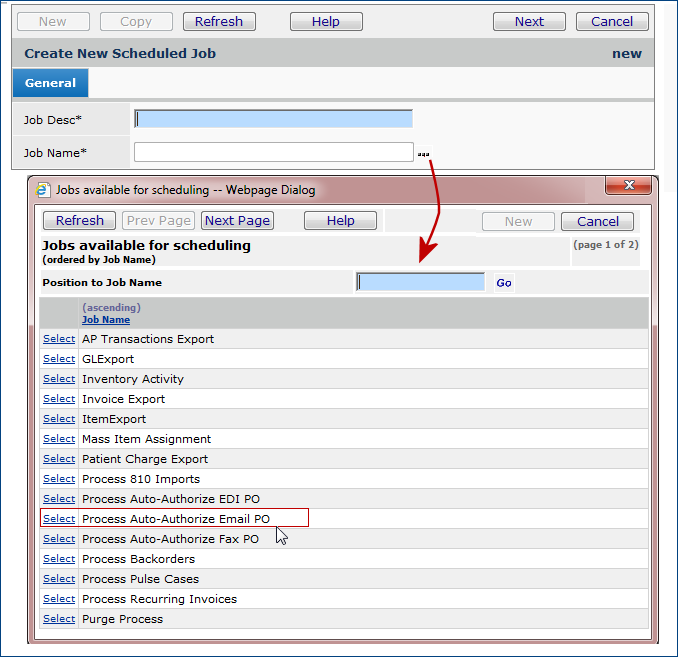In this screenshot, we see a user interface of a scheduling program. At the top of the screen are several buttons labeled "New," "Copy," "Refresh," "Help," "Next," and "Cancel." Below those buttons is a header that reads "Create New Scheduled Job." Beneath this header, there's a prominent blue button labeled "General."

Further down, there's a field labeled "Job Description" for entering a job's description, and below that is another field labeled "Job Name." Moving even further down, there's another section titled "Jobs Available for Scheduling Webpage Dialog," which includes buttons for "Refresh," "Previous Page," "Next Page," "Help," "New," and "Cancel."

The section also contains another header, "Jobs Available for Scheduling," followed by the instruction "Position to Job Name." Below this instruction, there is a list of job names. The job names listed from top to bottom are:

1. AP Transactions Export
2. GLE Export
3. Inventory Activity
4. Invoice Export
5. Item Export
6. Mass Item Assignment
7. Patient Charge Export
8. Process A10 Imports
9. Process Auto Authorized EDI PO
10. Process Auto Authorized Email PO (highlighted in a red square).